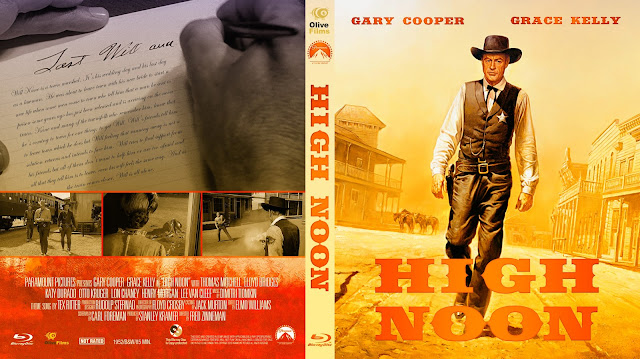This image displays the front and back covers of a DVD case for the movie "High Noon," laid out flat to reveal all sides. On the left side, the back cover features an image of hands writing or signing, accompanied by three smaller illustrations that appear to be scenes from the movie. Below these illustrations, the background transitions to a reddish-orange color, listing the names of actors, producers, and other credits typical of a film's back cover. The spine of the DVD case, positioned vertically in the center, prominently displays the title "High Noon" and includes the Paramount icon at the top.

The right side presents the front cover, with the title "High Noon" written in large capital orange letters across the bottom. Above the title stands a man clad in Western attire—a dark brown vest, dark brown pants, and a white long-sleeve shirt—complemented by a sheriff's star on his vest and a dark brown cowboy hat atop his head. The scene behind him depicts an old Western town with historic buildings and horses further enhancing the theme. At the top of the front cover, the actors’ names are displayed: "Gary Cooper" on the left and "Grace Kelly" on the right.

Overall, the intricate design and detailed elements of this DVD case emphasize the classic Western aesthetic of "High Noon," encapsulating the essence of the movie.